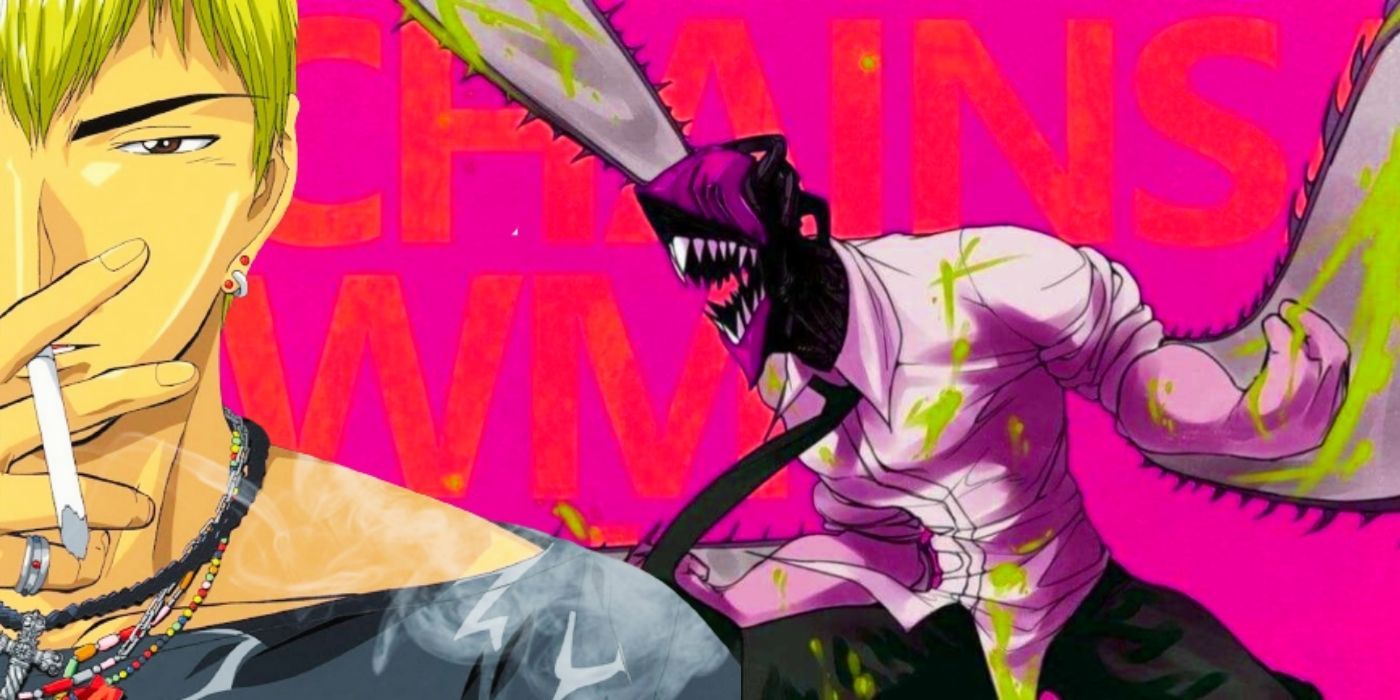In a vibrant anime-style drawing, the left side of the image features a man with neon yellow, straw-like hair forming a widow’s peak, and thick black eyebrows. He is smoking a cigarette and wears a black choker necklace, a gray off-the-shoulder top, and multiple other necklaces. The background is a bold magenta with reddish-orange letters reading "chainsaw man."

On the right side of the image stands a menacing creature with the body colored in shades of purple and black, white sharp teeth, and chainsaws attached to both its head and arm. The monster also dons a white button-down shirt splattered with green liquid and a black tie, complemented by black pants. The detailed, chaotic composition captures the surreal and intense nature of the scene.